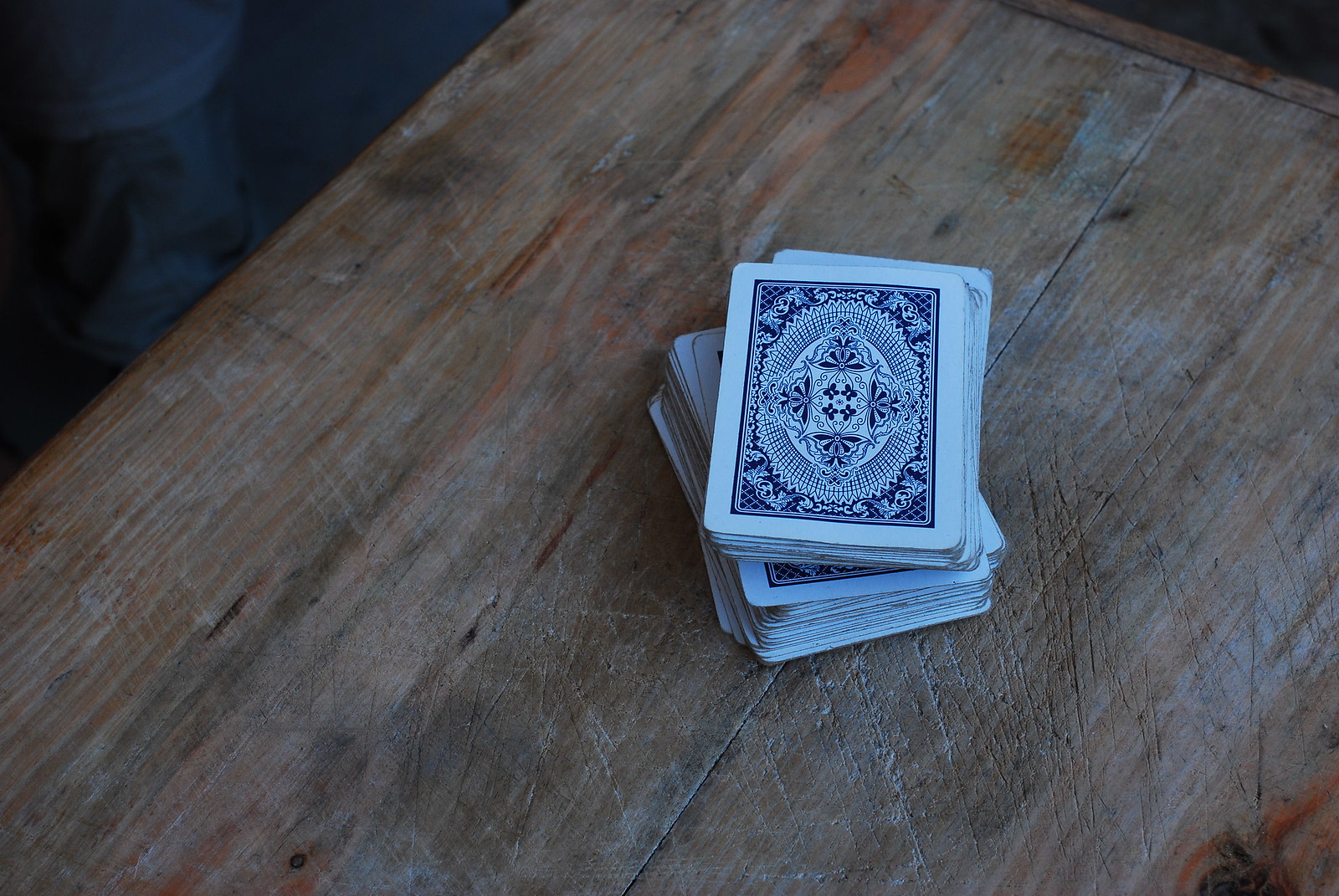A stack of playing cards sits on a worn wooden table or bench. The surface of the wood is light brown and grey with numerous cut marks, suggesting it has been used as a cutting board. In the image's top-left corner, there's a glimpse of dark fabric, possibly a pant leg, set against a dim background. The playing cards are imperfectly stacked at the center of the image, with a slight tilt about three-quarters of the way up. The cards are face down, showcasing an intricate blue and white ornamental design on their backs. This design features a central square surrounded by complex patterns of lines and markings.